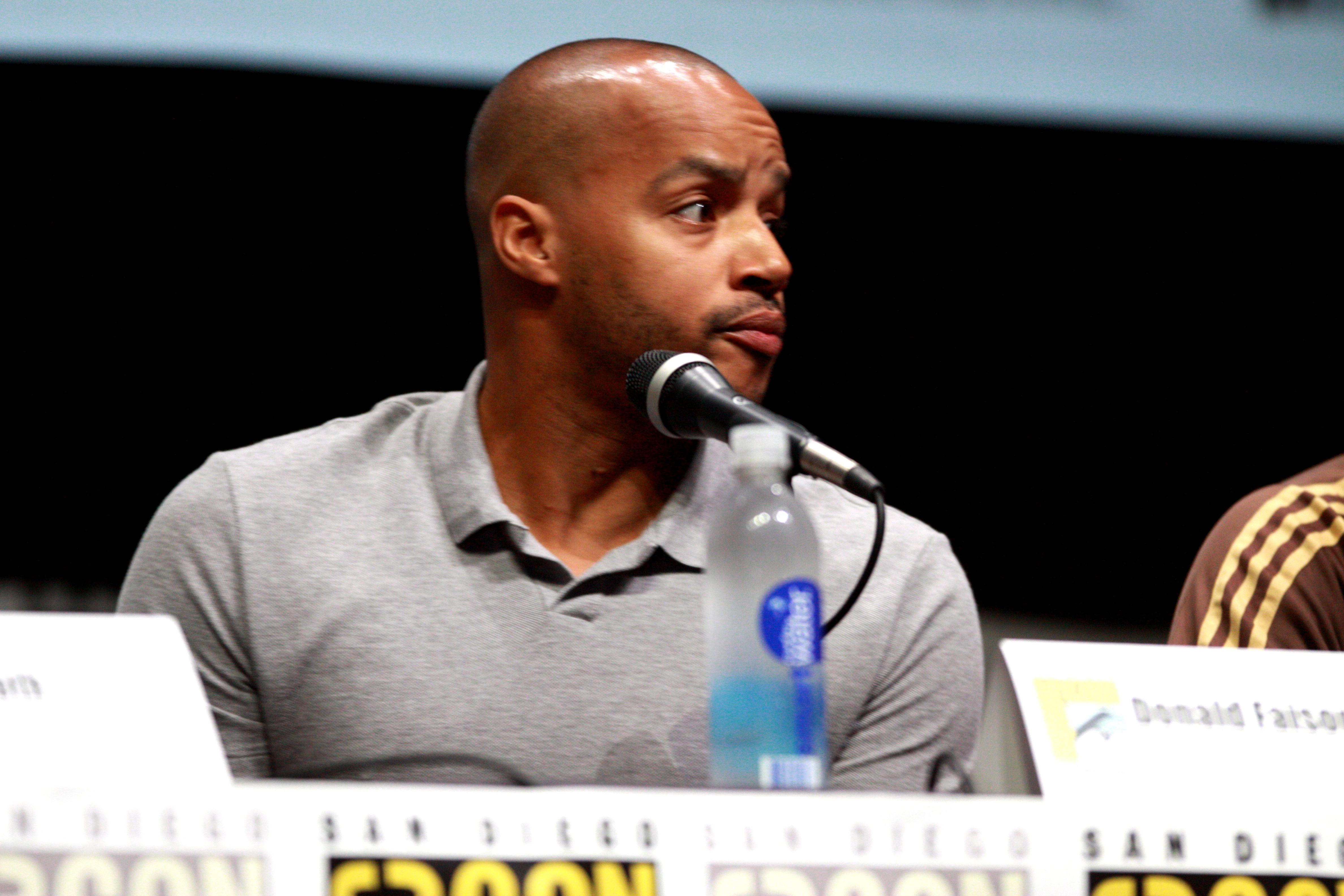This image captures an African-American male actor, Donald Faison, well-known for his role in the TV show "Scrubs," during a Comic-Con event in San Diego. He is seated and facing forward, with his head turned slightly to the right. Donald is wearing a gray, collared polo shirt and is bald with a shiny dome, sporting a faint beard and mustache. In front of him is an unopened bottle of Smartwater, identifiable by its clear cap and distinct blue and white label. A microphone is also positioned before him, though he appears to be looking away, not speaking at the moment. The background is primarily black, with a partial glimpse of a projector screen at the top. To his right, part of another person's shoulder is visible, clad in a brown shirt with yellow stripes on the sleeves. The iconic Comic-Con San Diego logo is horizontally positioned at the bottom of the image.